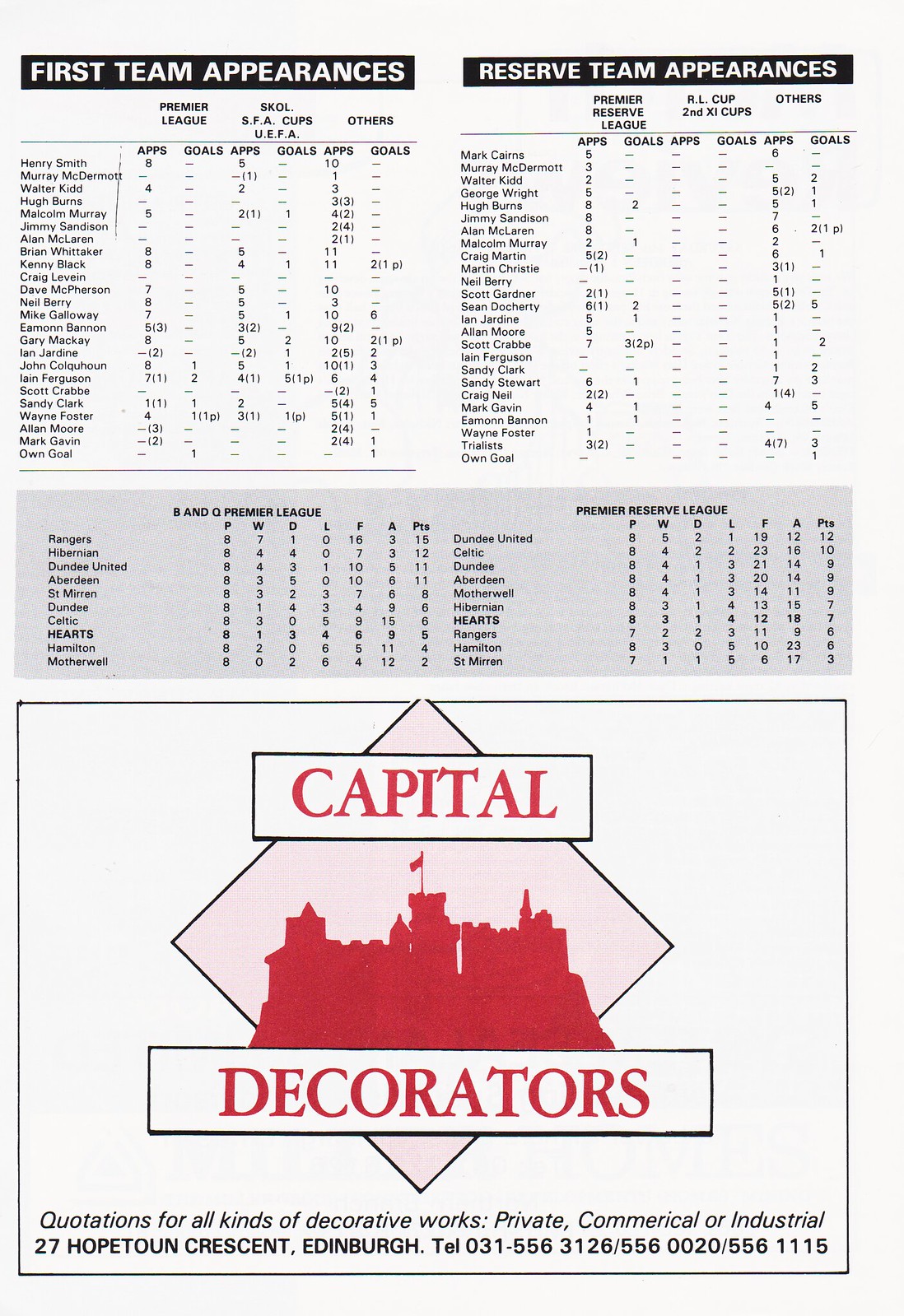The image is a detailed sports team roster poster, primarily focusing on professional soccer in Europe. It is divided into two main sections with headers: "First Team Appearances" on the left and "Reserve Team Appearances" on the right. Each section lists players along with their statistics, including appearances (Apps) and goals (Goals) for different competitions such as the Premier League, SKOL, SFA Cups, UEFA, and others. The statistics are organized in a structured manner with black banners and white text. The main color scheme of the poster is white, black, and red.

Beneath the players’ statistics, a significant portion of the poster is dedicated to an advertisement for Capital Decorators, a company offering quotes for various decorator works including private, commercial, and industrial projects. The advertisement includes the company's logo, which features a red castle within a rotated pink diamond, and provides contact information with their address at 12 Hope Tune Crescent, Edinburgh, Great Britain, alongside a telephone number. The overall design lacks any images of people or animals, focusing solely on the textual information and advertisement.